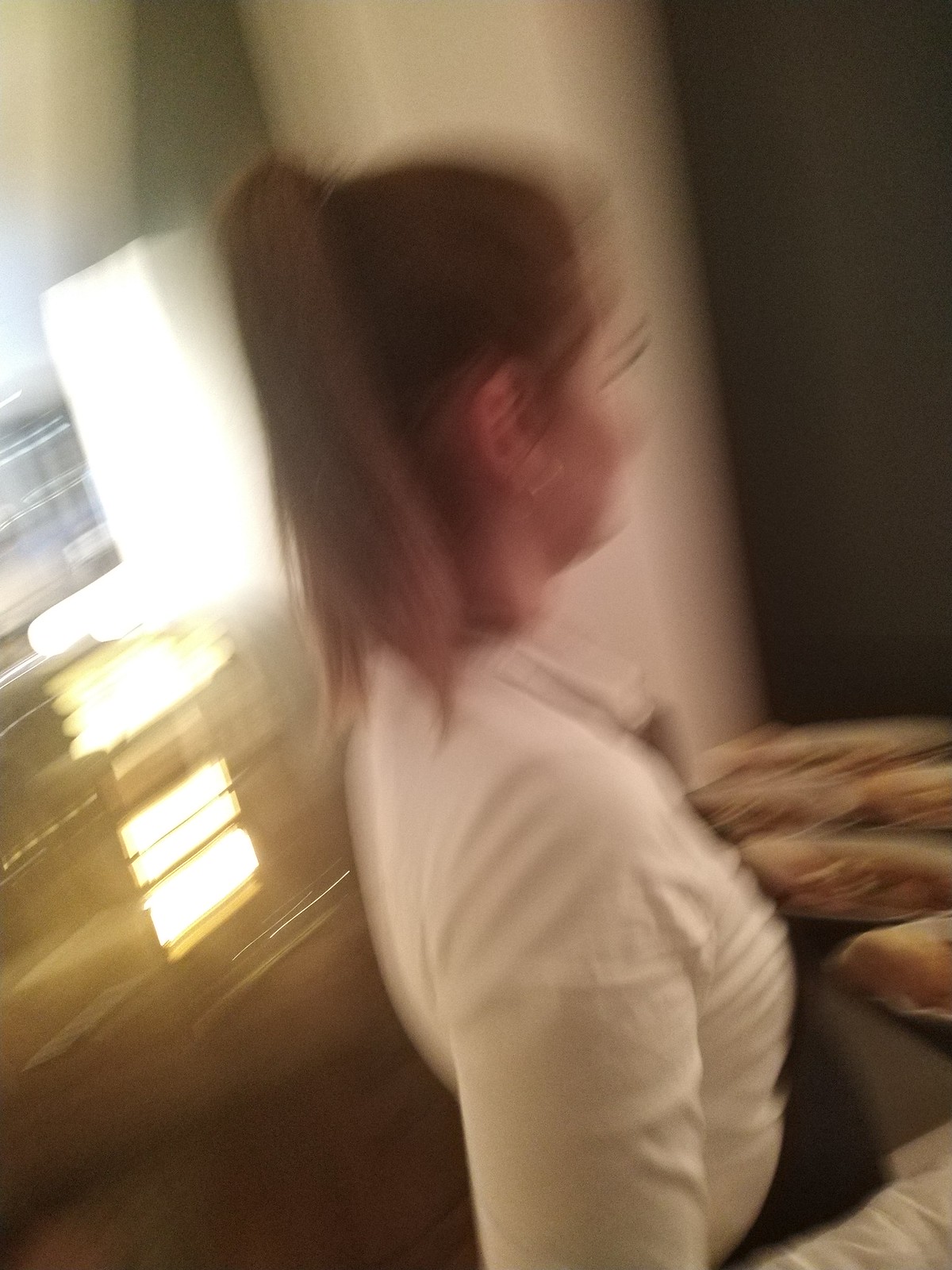In the center of the image, a person with a ponytail and long eyelashes is featured. They are wearing a white shirt and a distinctive brunette-colored, wrinkled earring. The person appears to be holding a plate of food or multiple dishes, although it is slightly out of focus. The background includes a wall that is darker on the right side and transitions to a lighter white on the upper left. An open doorway on the left side allows light to stream in. Additionally, there is a window on the left with some sort of bars, also letting in light. The floor in the scene appears to be dark.